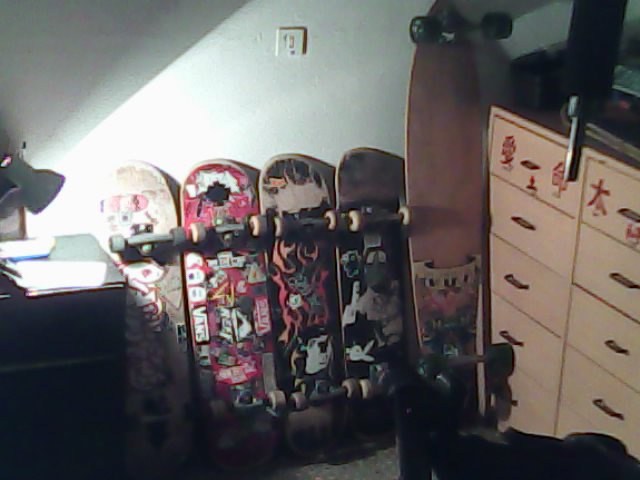This photograph captures the interior of a bedroom where five skateboards lean against a white or light blue wall, illuminated by a small white desk lamp perched on a cluttered table to the left. The skateboards, featuring varied graphics and stickers, appear well-used with worn-down tails, indicating they belong to an avid skateboarder. Among them, four are of regular size and heavily adorned with bright stickers, whereas the fifth board, positioned on the right, is a significantly longer longboard with a classic surfboard shape, sporting large wheels and wide trucks but devoid of any stickers. To the left of the skateboards is a small desk, and on the right, a peach-colored tall dresser with Chinese characters on it and wooden handles, possibly used for clothing. The room otherwise lacks a visible light source, with the lamp being the primary illumination, casting a focused glow on the skateboards.